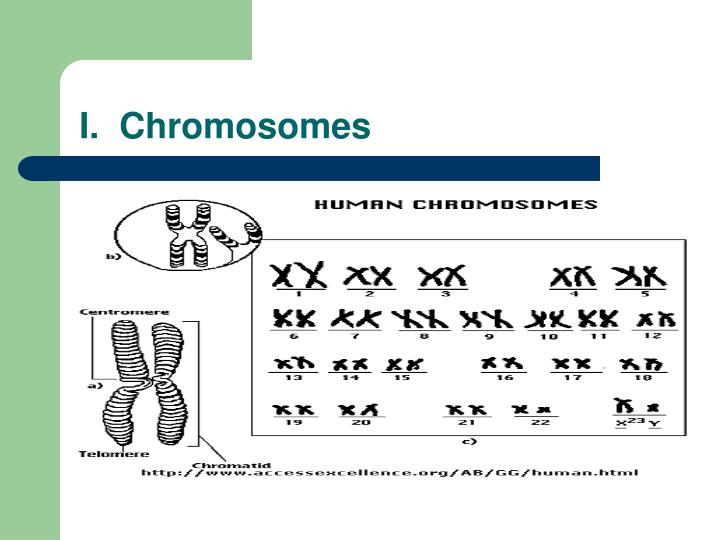The image is a detailed scientific diagram focusing on chromosomes, resembling a page from a textbook or manual. The central theme is showcased prominently with a green title reading "1. Chromosomes" at the top, followed by a horizontal blue bar and the phrase "Human Chromosomes" in black capital letters below it. The layout is clean, set against a white background with a decorative green border along the entire left side.

Prominently featured in the diagram are two images on the left side: the first is a circular depiction of a chromosome pair in an X-shape, and the second is an enlarged, detailed view of this pair, with annotations identifying various parts of the chromosome, though the text is hard to read. 

To the right, a partitioned square with black trim displays 23 pairs of chromosomes, neatly organized with X shapes corresponding to each number, from 1 to 23, to illustrate human chromosomal pairs.

At the bottom of the diagram, additional information can be accessed via a URL, which reads http://www.accessexcellence.org/abgg/human.html.